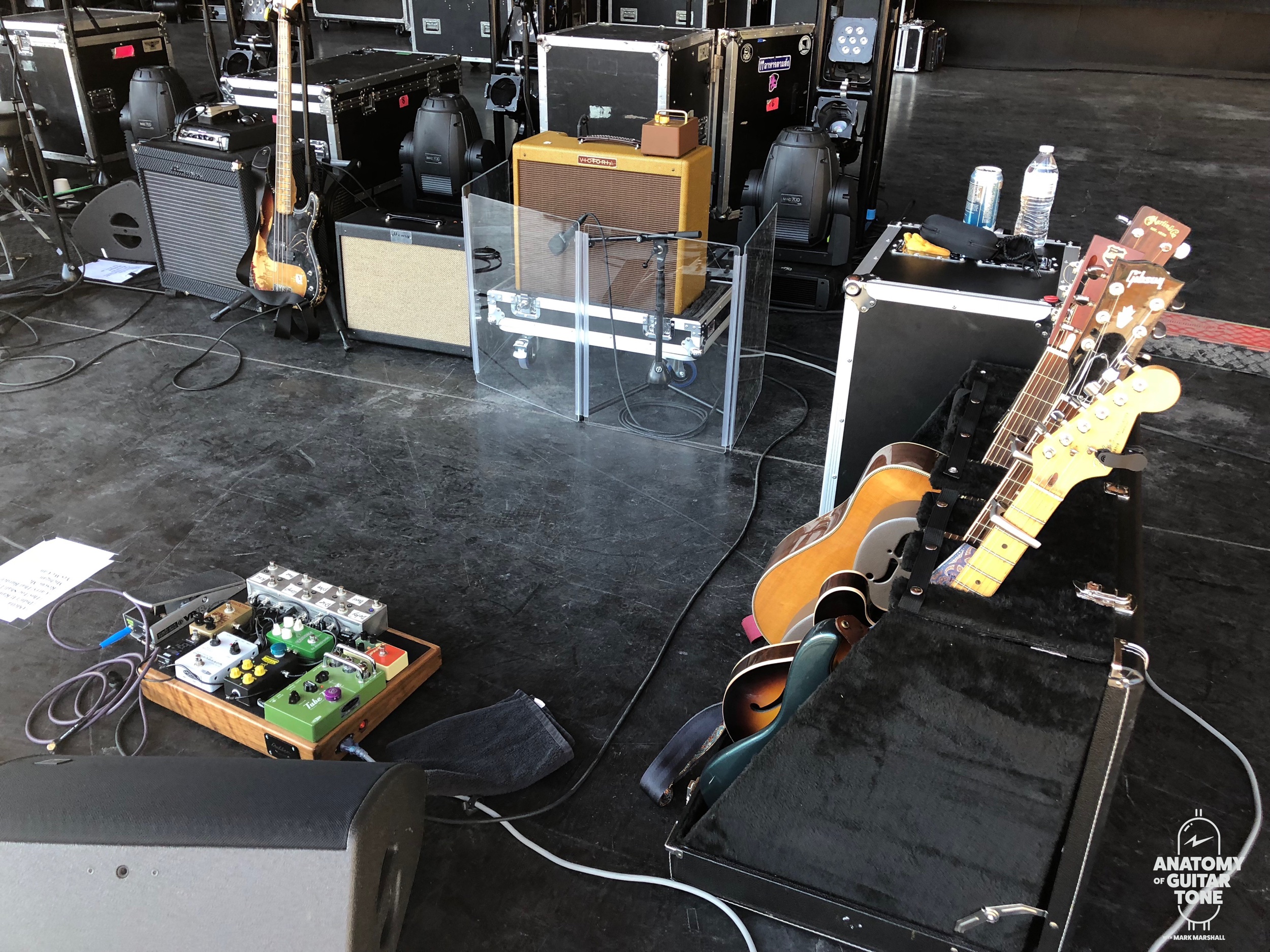The image depicts a detailed and photorealistic scene of a sound studio filled with an array of musical equipment, almost looking like a stage setup ready for a concert. Multiple electric guitars, both black and orange, are prominently featured, some resting in stands, while others are connected to various amplifiers and sound boxes. These amplifiers, stacked in several locations around the studio, exhibit a range of sizes and colors, including human-sized stacks in the top left and more in the far distance. One notable amplifier has a bottle of water and an energy drink perched on top of it, indicating a musician's presence. At the center-left on the floor lies a complex pedalboard with various diodes of different colors, connected via wires to an amplifier, used for altering guitar tones. The floor boasts a smooth, matte black concrete finish, matching the room's overall dark aesthetic, which is further emphasized by the black walls. In the bottom right corner, there is a caption that reads, "Anatomy of Guitar Tone," summarizing the focus on the intricacies of developing guitar sounds. Despite the room's apparent bustling activity, there's an underlying sense of order and purpose, with all instruments and equipment meticulously arranged as if preparing for a performance, yet no musicians are present in the scene.